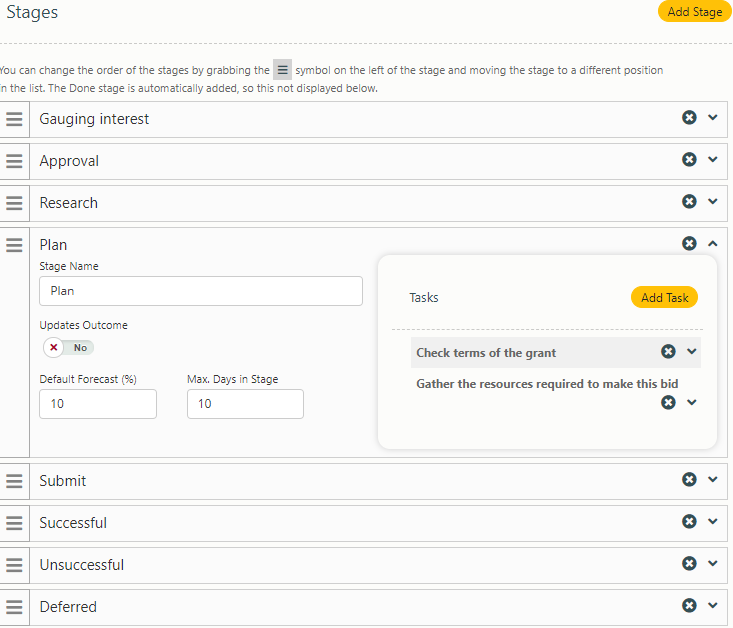The image depicts a web page with a white background and black text detailing a workflow management interface. 

At the top-left corner of the page is a section labeled "Stages," while the top-right corner features a yellow button labeled "Add Stage." Beneath this header, an instructional note explains that users can rearrange the order of stages by dragging the menu symbol on the left next to each stage. It also mentions that the 'Done' stage is automatically added and thus not displayed below.

The page further contains drop-down menus for different stages, including "Gauging Interest," "Approval," and "Research." One drop-down menu, labeled "Plan," is currently open, providing additional details:
- Stage Name: Plan
- Update Outcomes: Click to know
- Default Forecast: 10
- Max Days in Stage: 10

To the right, there is a pop-up box labeled "Task," showing an "Add Task" section with tasks such as "Check terms of the grant" and "Gather the resources required to make this bid," each accompanied by their respective drop-down menus.

Further down, there are drop-down menus for different outcome stages including "Submit," "Successful," "Unsuccessful," and "Deferred." Each of these boxes includes a close button.